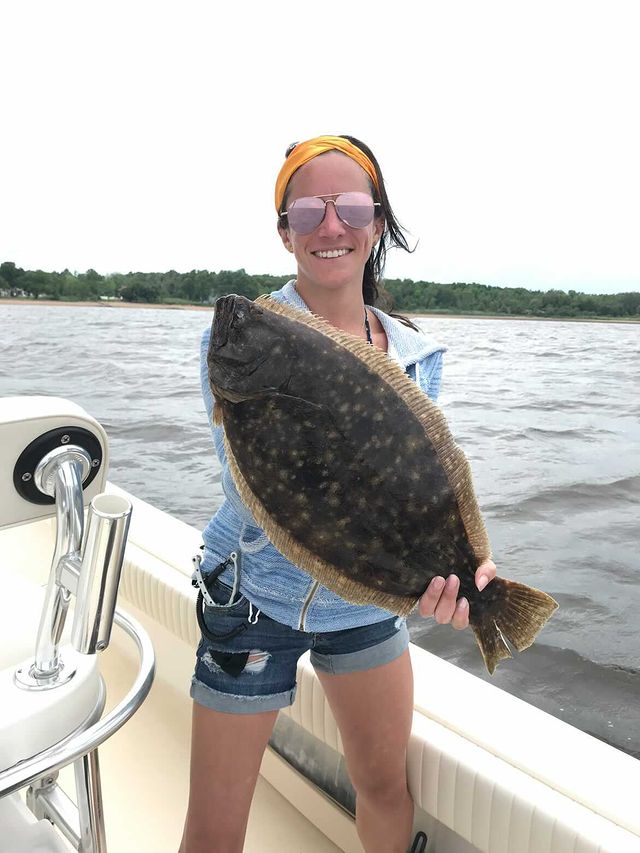In this image, a fit, smiling woman is standing on a white boat, proudly holding a large, flat, dark brown fish speckled with greenish and lighter brown spots. The fish is as long as her chest, with prominent spike-like dorsal and lower fins. She grasps the fish by its tail with her left hand, while its tightly closed mouth points downward. The woman is dressed in rolled jean shorts and a light blue zipped-up hoodie. Her long brown hair is pulled back with a yellow headband, and she wears dark-tinted sunglasses. Behind her, a body of water stretches to a distant shoreline, featuring a mix of wooded areas and a few houses on the left. The white sky fills the upper part of the image, creating a serene backdrop for this triumphant moment.